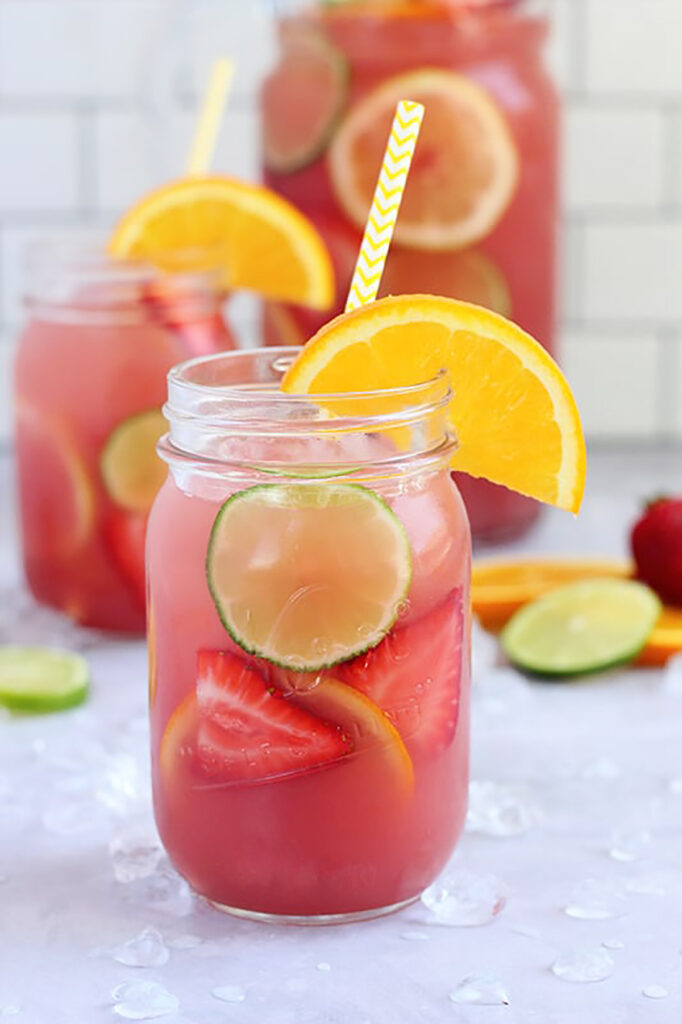In this close-up photograph taken indoors, two mason jars sit on a white surface, each filled with a vibrant pink liquid that appears to be a refreshing beverage. Both jars contain slices of lemon and orange, with additional halves of strawberries visible through the clear glass. Garnishing the rim of each jar is a slice of orange. A yellow and white striped straw is inserted into each jar. The surface around the jars is dotted with a few clear droplets, suggesting condensation or spillage. 

In the foreground, the jars are sharply in focus, while in the background, a larger, slightly blurry jar can be seen. This larger jar, decorated with slices of lemon and lime, hints at being a ceramic or jug-like container holding more of the same pink drink. The backdrop of the image is a clean, white tiled wall, reminiscent of subway tiles, adding a minimalist and modern touch to the overall setting.